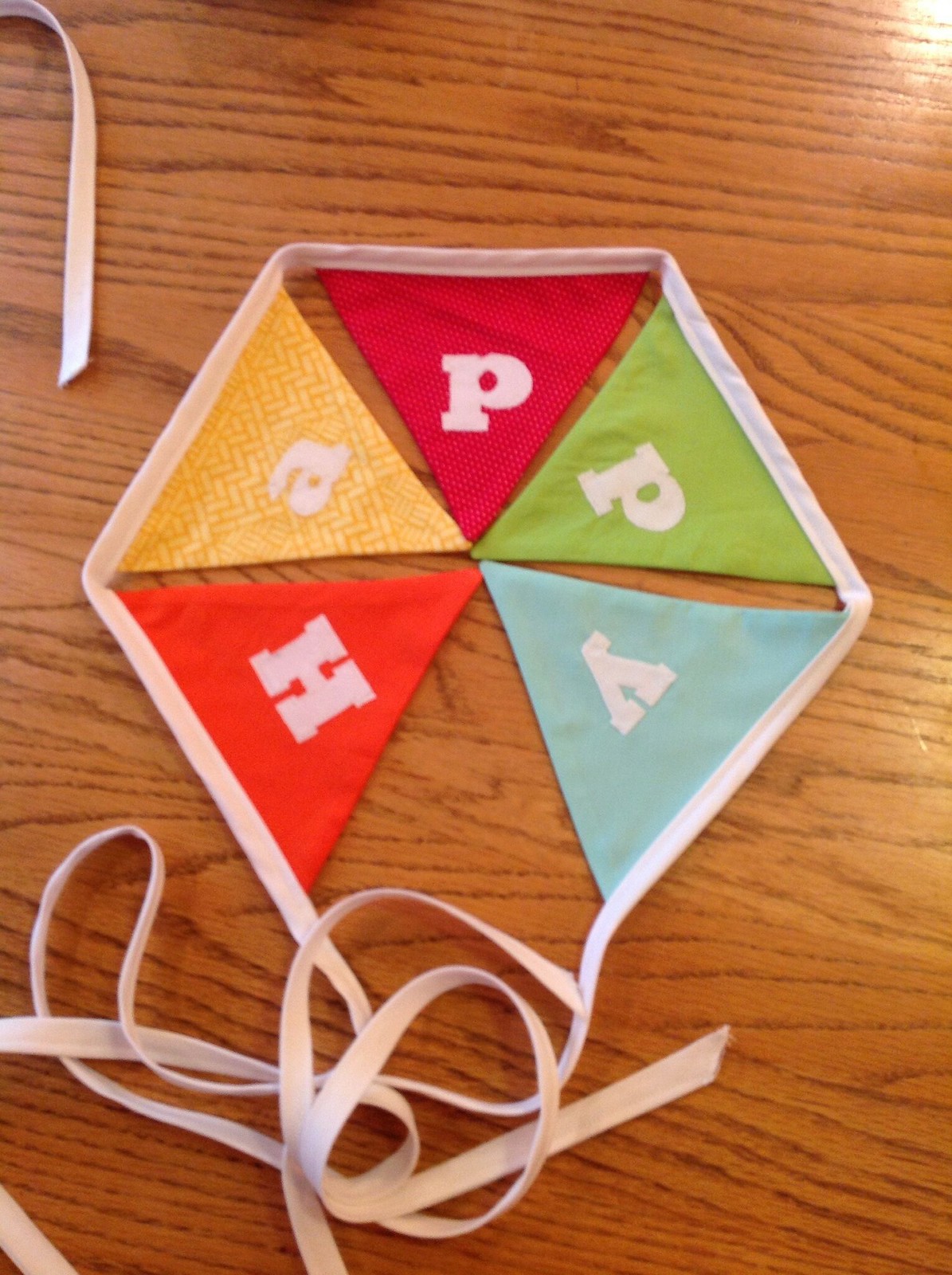This photograph captures a festive fabric banner laying atop a wooden table, with sunlight streaming in from the top right corner. The banner, designed to spell "happy," features a series of colorful triangles, each adorned with a white letter. The triangular pieces form a near-hexagonal shape, with five sides filled and the sixth side left open, partially due to the coil of excess string at the bottom.

Starting from the bottom left and moving clockwise, the first triangle is orange with an uppercase "H," followed by a yellow triangle with a lowercase "a" and a darker zigzag pattern. Next is a red triangle with a lowercase "p" dotted pattern, then a green triangle with another lowercase "p," and finally a light blue triangle with a lowercase "y."

Each end of the banner is equipped with strings for tying. In the top left corner of the image, a hint of another string suggests the presence of a second banner, possibly bearing the rest of a celebratory phrase such as "birthday." The intricate details and vibrant colors of the banner make it a charming focal point against the rustic wood grain background.